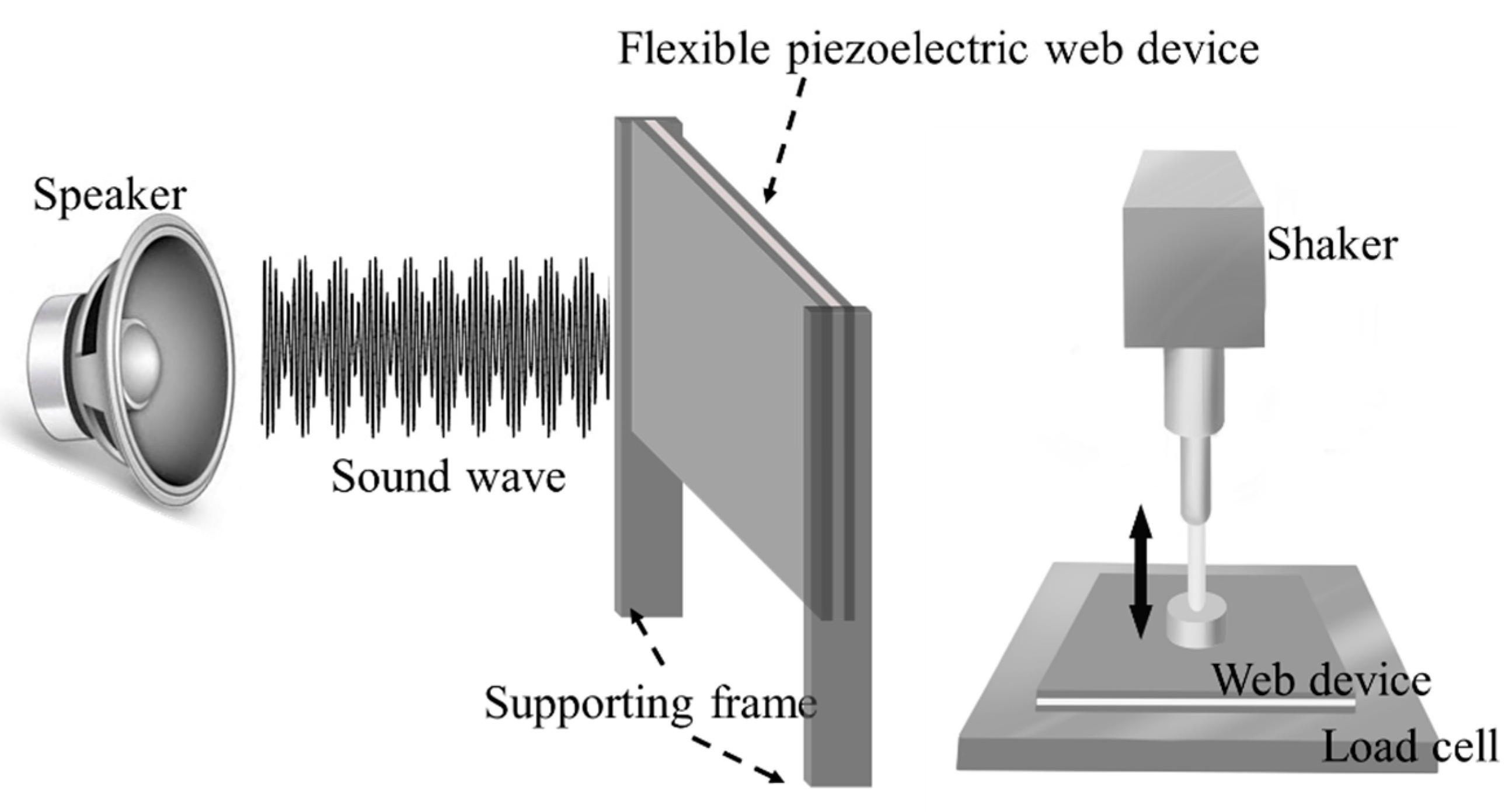This diagram illustrates the components and functioning of a Flexible Piezoelectric Web Device, depicted in grayscale with detailed labels. Starting from the left, a 'speaker' emits 'sound waves' shown as a series of wave illustrations. These waves travel towards a 'supporting frame,' which is visually similar to a billboard with two posts and a flat section between. Adjacent to this, the 'Flexible Piezoelectric Web Device' is highlighted, where sound waves interact. Positioned to the right, a 'shaker' device is depicted pressing down on the web device, with an arrow indicating an up-and-down motion labeled 'web device load cell.' The entire layout features clear text annotations and directional arrows, providing a comprehensive understanding of the setup and interactions.